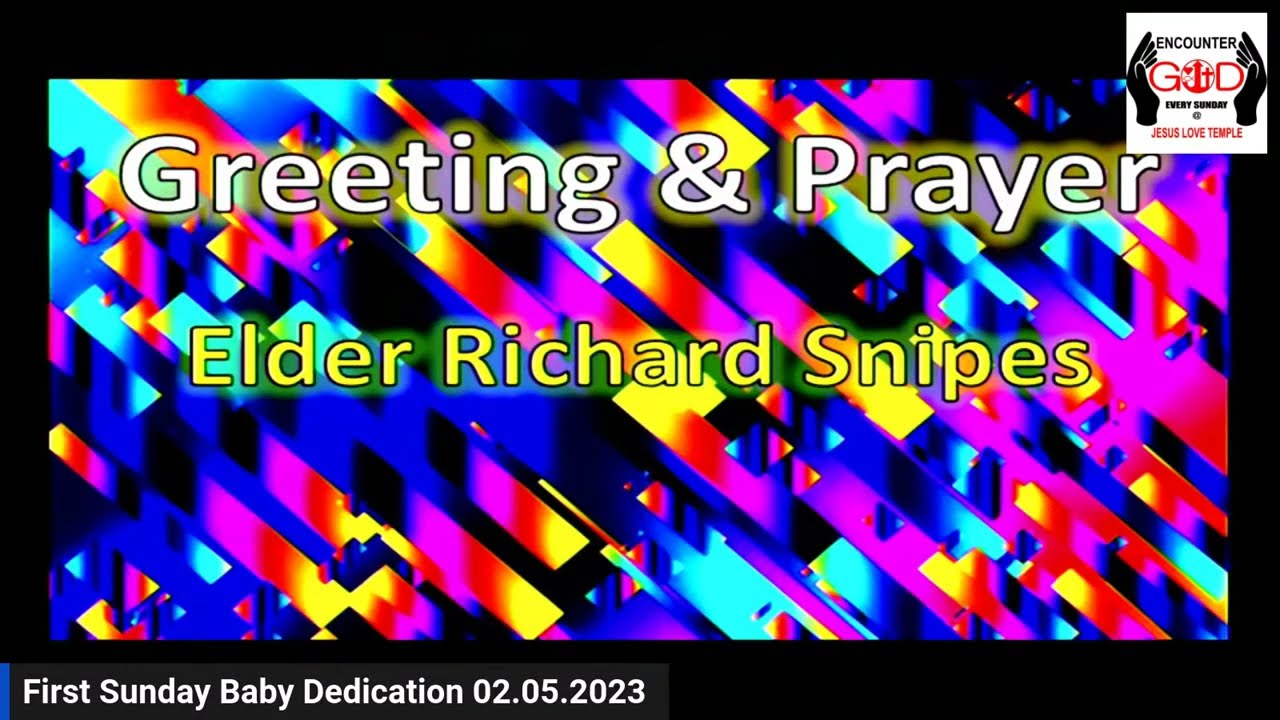The image is a vibrant and colorful advertisement with a black border surrounding it. The background features thick, diagonal stripes in bright, glowy colors such as pink, black, yellow, red, and blue, creating an abstract style. At the top center, the words "Greeting and Prayer" are displayed in white font with a green outline. Just below, the text "Elder Richard Snipes" appears in yellow font with a black border. In the bottom left corner, a gray rectangular box contains the text "First Sunday Baby Dedication 02.05.2023" in white font, with each word capitalized. The upper right corner of the image features a logo with the words "Encounter God Every Sunday Jesus Love Temple," accompanied by a symbol of two hands on either side of the word "God." Inside the letter "O" of "God" is a cross along with a couple of other icons. A small blue stripe is also visible in the very bottom left corner.